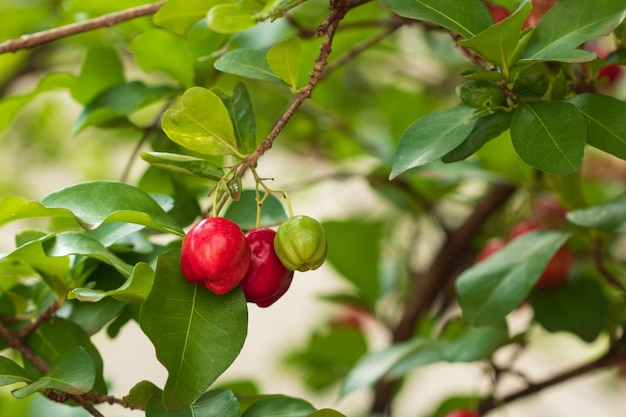This image showcases a tree branch prominently in the center, featuring a lush array of leaves and multiple fruits. On the highlighted branch, there are three distinguishable fruits: two are red and the third is green, with the green fruit being noticeably smaller. Additional red fruits are also present, extending to the right side of the plant and into the background, albeit less sharply focused. The fruits are reminiscent of small apples or perhaps berries, though their exact identity is unclear. The overall scene is rich with foliage, though some of the surrounding leaves and fruits are blurry, emphasizing the clarity of the central branch and its vibrant fruit. The ground is also slightly visible in the blurred background. Although the fruits might look tempting, their edibility is uncertain, resembling a cross between little tomatoes and peppers, and could potentially be unfit for consumption.